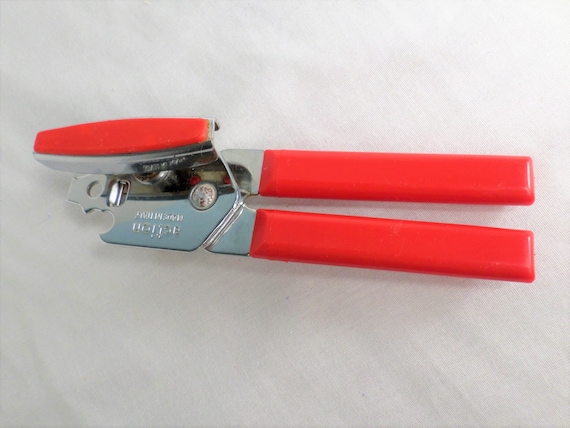A hand-held, hand-operated can opener is prominently displayed on a gray surface, which transitions from a darker shade on the bottom left to a lighter tone as it moves to the upper right. The can opener features distinct dual handles on the right side, covered in a rubbery, dark orange or light red material. These rectangular handles catch the eye with highlights of white light reflecting off their edges. Central to the design is a chrome hinge, polished to a silver shine, marked by a prominent dot at the middle where its bolt or rivet is located, allowing the handles to open and close. 

On the left side, beyond the handles, the body turns metallic chrome. A turning knob projects straight up from the handle, topped with the same orange stripe as the handles, enhancing its cohesive appearance. Visible on the bottom left corner of the device is a half-circle design with two gripping points made for secure lid engagement. Additionally, there is a bottle cap opener feature integrated into the lower left chrome section, identifiable by its hook-like form that fits under the lip of a bottle cap for manual opening. The overall composition presents a meticulously detailed image of a versatile kitchen tool.